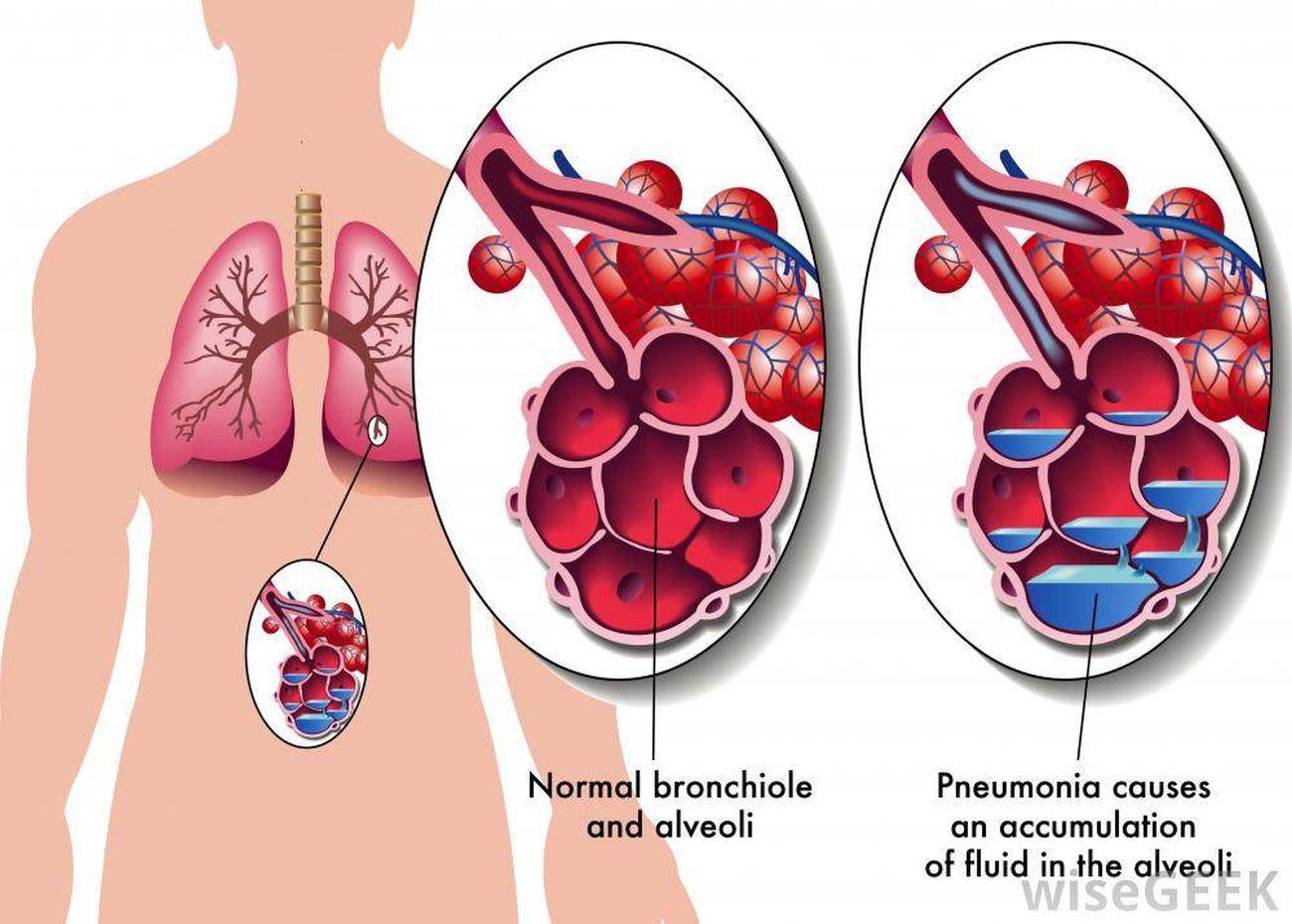This detailed medical diagram illustrates the human lungs and the impact of pneumonia on the bronchioles and alveoli. On the far left, the image features a silhouette of a man's upper body from his chin to his waist, showcasing a pair of lungs inside. Positioned within the lungs, there is a small inset pointing to a branching area of the bronchioles. This inset is magnified into two larger oval blow-ups to the right.

The first oval, labeled "normal bronchiole and alveoli," depicts healthy lung structures resembling a raspberry on a stick, with small red alveoli. Adjacent to this, the second oval illustrates a similar structure but with blue alveoli indicating pneumonia. The caption here notes that "pneumonia causes an accumulation of fluid in the alveoli." 

The color palette includes salmon pink for the body silhouette, with white, pink, red, blue, and gray dominating the lung illustrations. The setting suggests that this diagram is part of a medical educational presentation or resource. At the bottom right corner of the image, there is an attribution to Wise Geek, reinforcing its educational purpose.